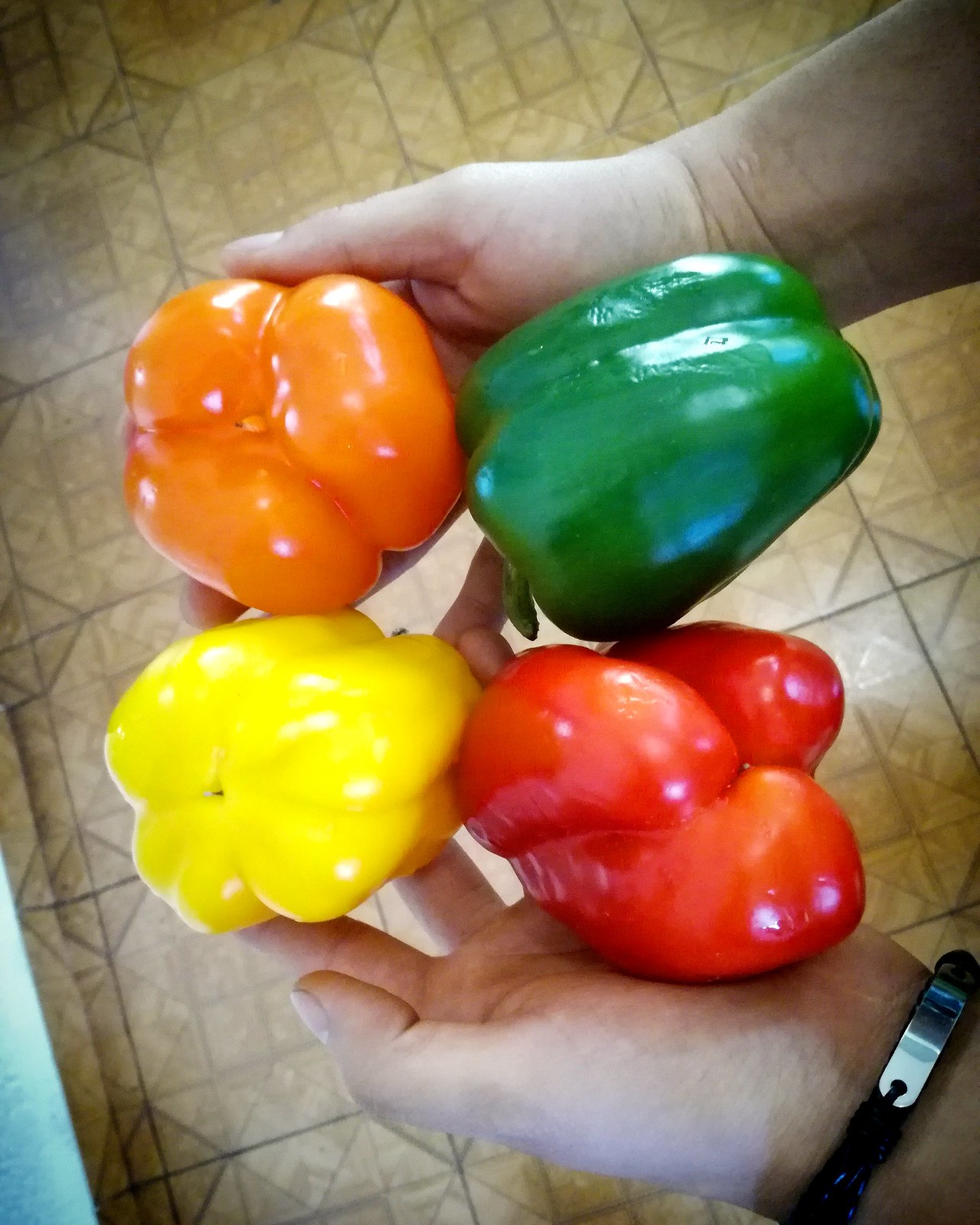In the photograph, a pair of male hands is holding four colorful capsicums—yellow, orange, green, and red. The red capsicum stands out with its asymmetrical shape. The hands, viewed from the palm side, reveal a black bracelet with a silver plate on the left wrist. The background features a well-worn linoleum floor with a dark tan, geometric square pattern, reminiscent of the 1970s. The lighting is subdued, possibly from a sunset. The person seems poised to cook something tasty, proudly presenting the vibrant peppers. The bottom view of the capsicums is visible, with the green one lying on its side, exposing its stem.